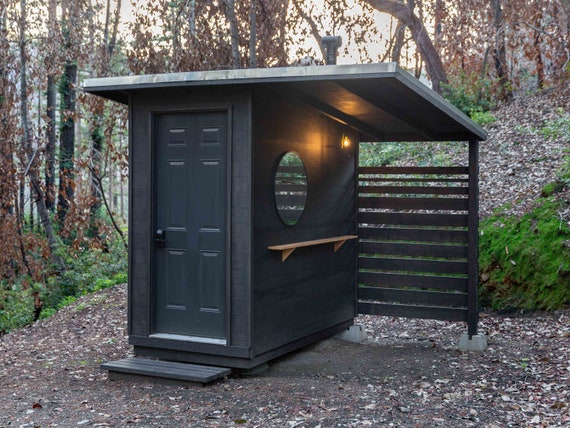In the serene autumnal forest, a modern outhouse stands, blending harmoniously with its natural surroundings. This small, rectangular structure is painted a dark color, possibly black or dark green, and is just a few feet wide and deep. Its dark blue, six-panel door with a black handle almost occupies the entire front width of the building. The sloping, lean-to roof adds a utilitarian charm, possibly made of tin or white material.

Situated at the base of a hill with mossy plants, the outhouse features a quaint, practical setup. On the right side, a circular mirror is mounted above a light brown wooden shelf, accompanied by a light bulb that casts an orange glow on the interior walls and roof. Adjacent to this, there's a small seating area shaded by an extension of the roof, providing a peaceful spot to rest.

The outhouse rests on a bed of brown dirt and fallen leaves, with towering trees showcasing amber foliage in the background. A lively green plant peeks from the bottom right, adding a splash of color to the earthy scene. This image vividly captures the blend of functionality and aesthetics in a rural, forested setting.